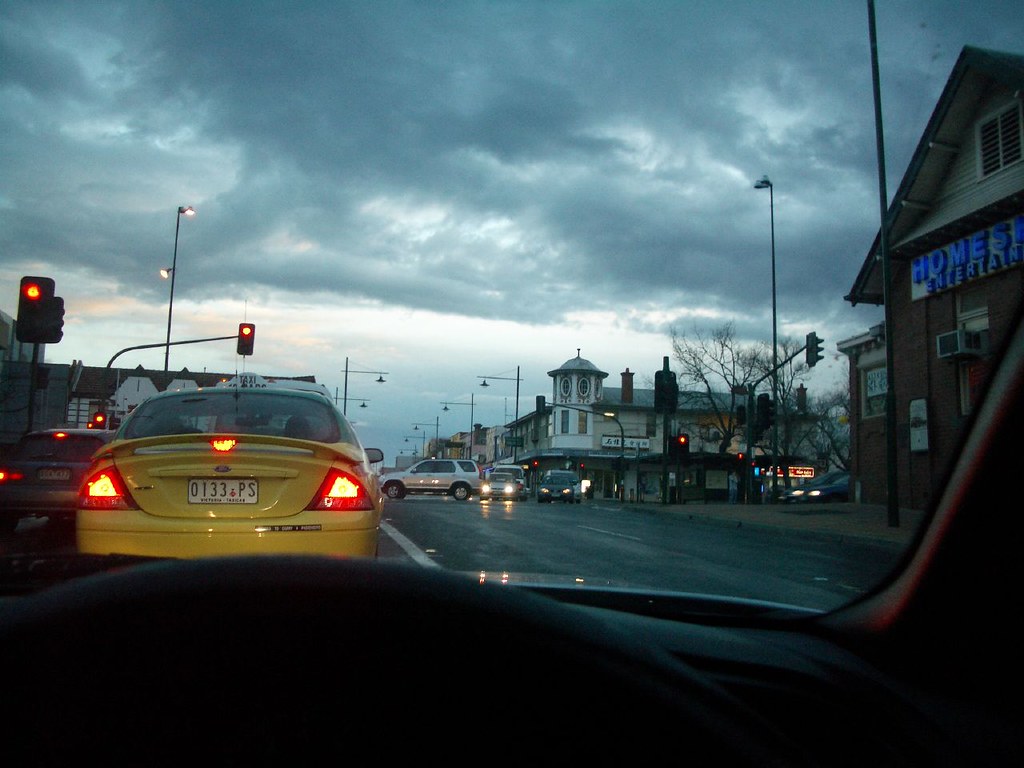The image captures a typical urban scene from the perspective of a passenger inside a car. The photograph is taken through the windshield, with the outline of the dashboard and steering wheel visible at the bottom of the image. Outside, a dark and ominous overcast sky looms, filled with light gray, dark gray, and almost black clouds, yet no rain has begun to fall as evidenced by the dry windshield. In the center of the image, a yellow car, possibly a taxi, with its brake lights on, sits at a red traffic light. Beside it is another car, bluish-green, heading left through the intersection. The streetlights on tall poles are lit, suggesting either early evening or late afternoon. To the right, a prominent two-story brick building with a peaked roof displays a blue lit-up sign reading "Homer's" or "HOME ENTERTAINMENT," and an air conditioner unit or camera protrudes from its side. Further in the distance, a leafless tree—indicating winter—stands next to another larger building, possibly a shopping center. Cars with their headlights on move in the background, illustrating typical city traffic.